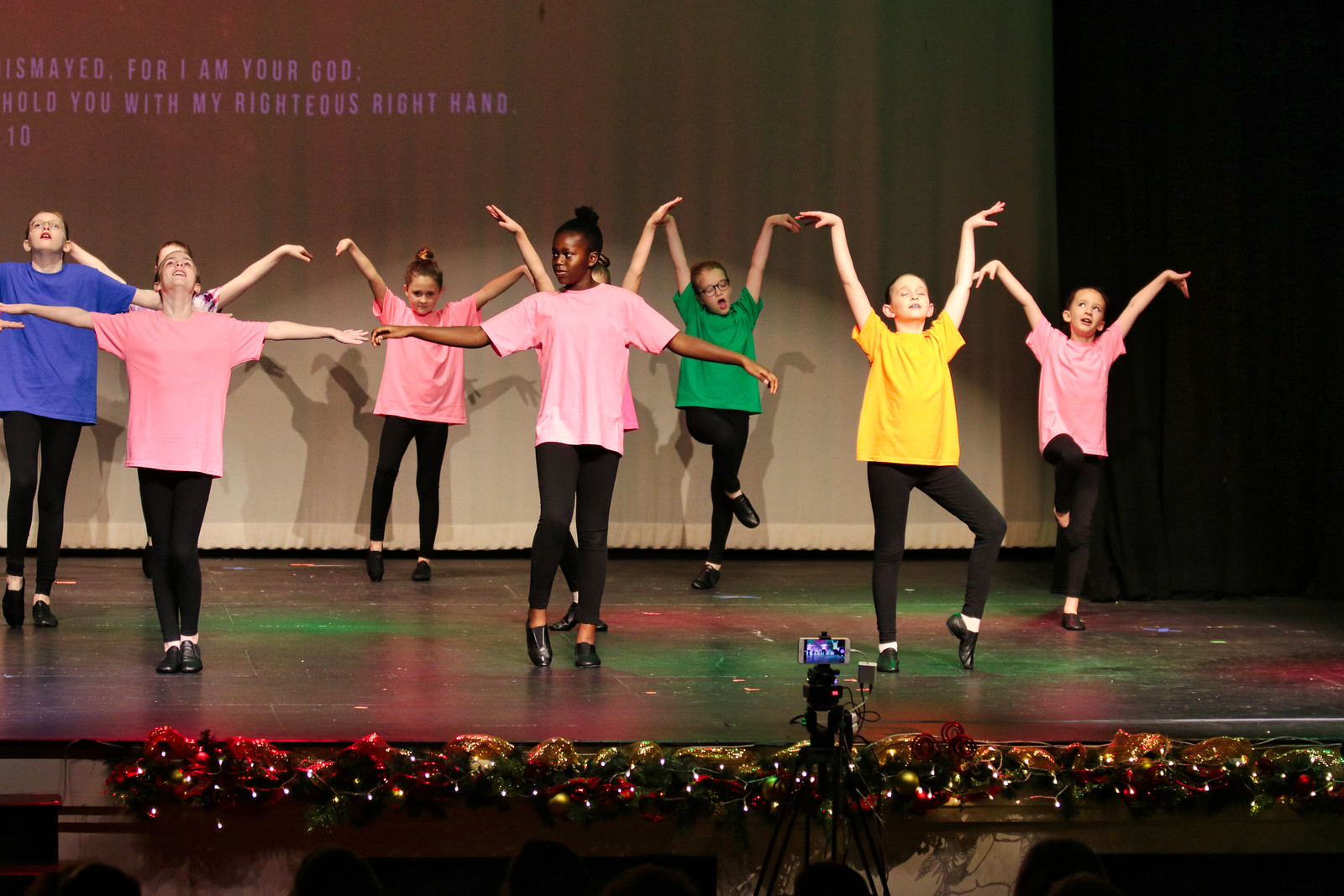In this detailed photograph of several young girls dancing on a large indoor stage with brown wood floors, the focal point is their synchronized dance performance. The girls, each wearing black tights and black tap dancing shoes, are dressed in colorful short-sleeved t-shirts – four in pink, one in blue, one in green, and one in yellow. They are spread across the stage horizontally, most with their arms raised or out to their sides, striking expressive poses.

Behind them, a large curtain with a spotlight beams a partially cut-off message: "dismayed for I am your God... hold you with my righteous right hand (Isaiah 41:10)." The stage is decorated with festive garland, bells, and holiday bows, suggesting a seasonal performance. Additionally, a camera is visible in the foreground, capturing their performance, alongside some Christmas lights adorning the edge of the stage. The overall setting is lively and vibrant, emphasizing the joyful spirit of the occasion.